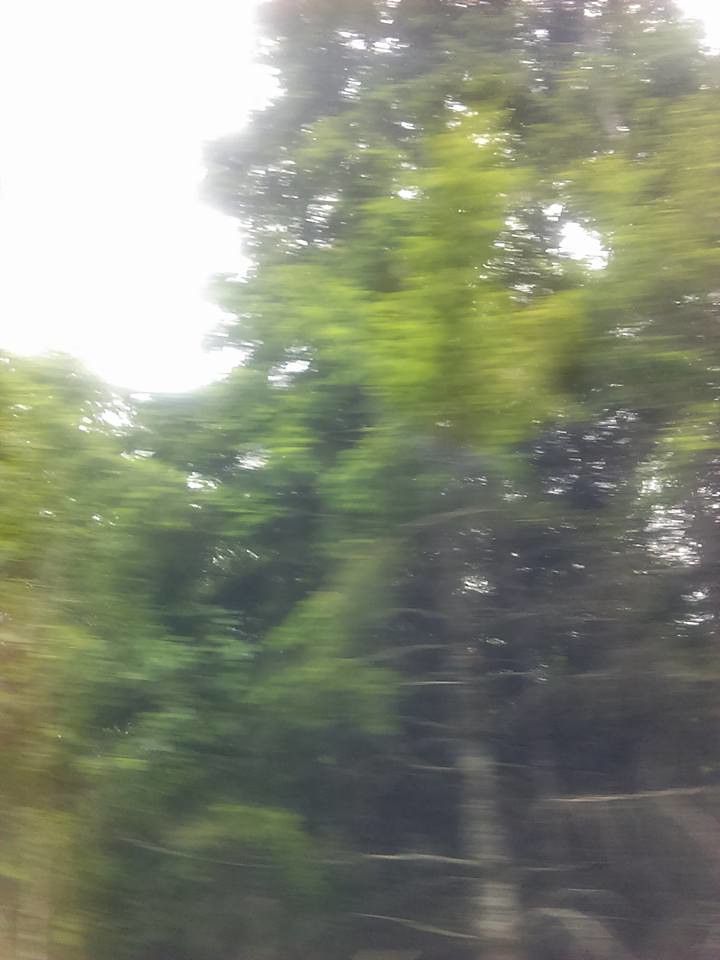In this photograph, a blur of motion creates an intriguing, albeit disorienting, view of a densely wooded area. The focal point is a large tree trunk in the foreground, standing tall with sparse leaves near its base and a thick canopy of green at its peak. Surrounding this main tree, a collection of tall, dark green trees extend upwards, their leaves blending into a luscious overhead cover. To the left, a shorter, bushy tree adds texture with its compact green foliage. The sky above is a bright, almost blinding white, illuminating the scene but washing out any details beyond the treetops. The forest floor at the bottom of the photo is a mix of brown dirt, grounding the image despite the blur that gives everything an impression of frenzied motion.